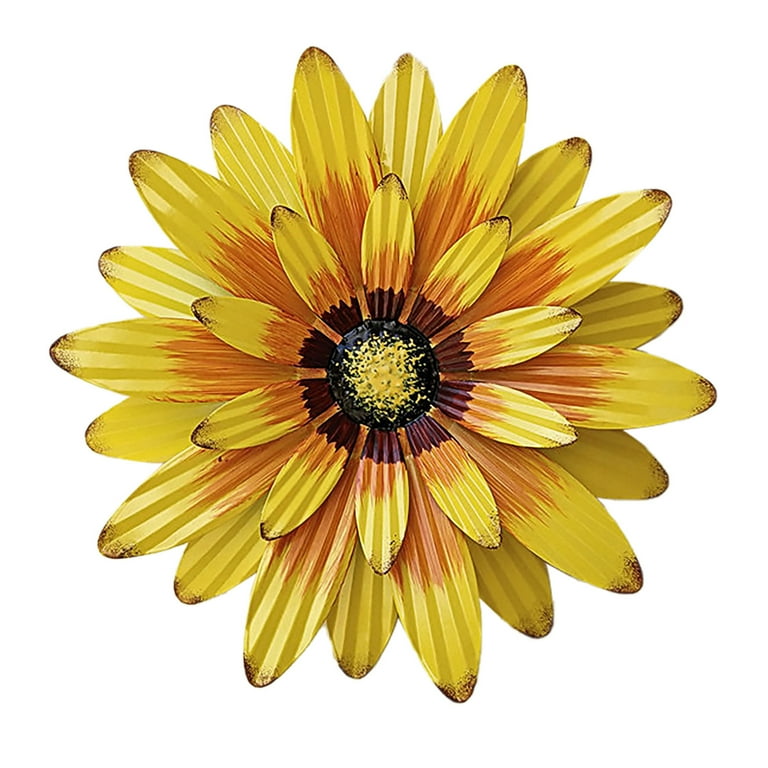This image depicts a metal sculpture of a large sunflower against a white background, emphasizing its intricate design and artistic details. The sculpture features three concentric layers of variegated petals, meticulously carved and painted in hues of yellow, orange, and red. The innermost layer boasts ten petals with a purple tint near the center. The center of the sunflower displays a rich black core with yellow speckled paint, circled by a ring of brown, a narrow band of orange, and then another layer of yellow, transitioning to brown speckles at the tips. This striking, three-dimensional art piece stands as a vivid focal point, with no stem visible, highlighting the beautifully curated layers and complex textures of the sunflower.